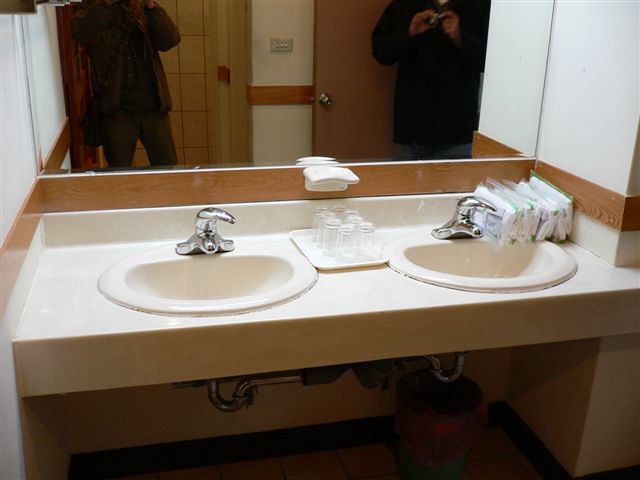This detailed photograph captures the vanity area of a bathroom, likely part of a hotel or public facility. The image shows a white counter with two identical ceramic sinks featuring silver faucets. These sinks appear to be oval-shaped with raised lips. Between them sits a tray holding eight small drinking glasses, all turned upside down. Additionally, there is a white porcelain soap dish on the tray. Against the back wall, on the right side of the counter, are several washcloths encased in plastic bags. 

A prominent large mirror with brown wooden trim at the bottom spans the width of the counter. Reflected in the mirror, we see a wooden door with a handle, a light fixture, and a white wall with a brown border. Also visible in the reflection are the torsos and legs, up to the knees, of two individuals dressed in dark clothing; one stands near the door while the other appears closer to the shower area that is tiled.

Underneath the counter, piping and plumbing fixtures are visible, adding to the utilitarian feel of the space. The visible wood molding for the backsplash enhances the simplicity of the design, suggesting that this bathroom is part of a modest, perhaps older establishment.